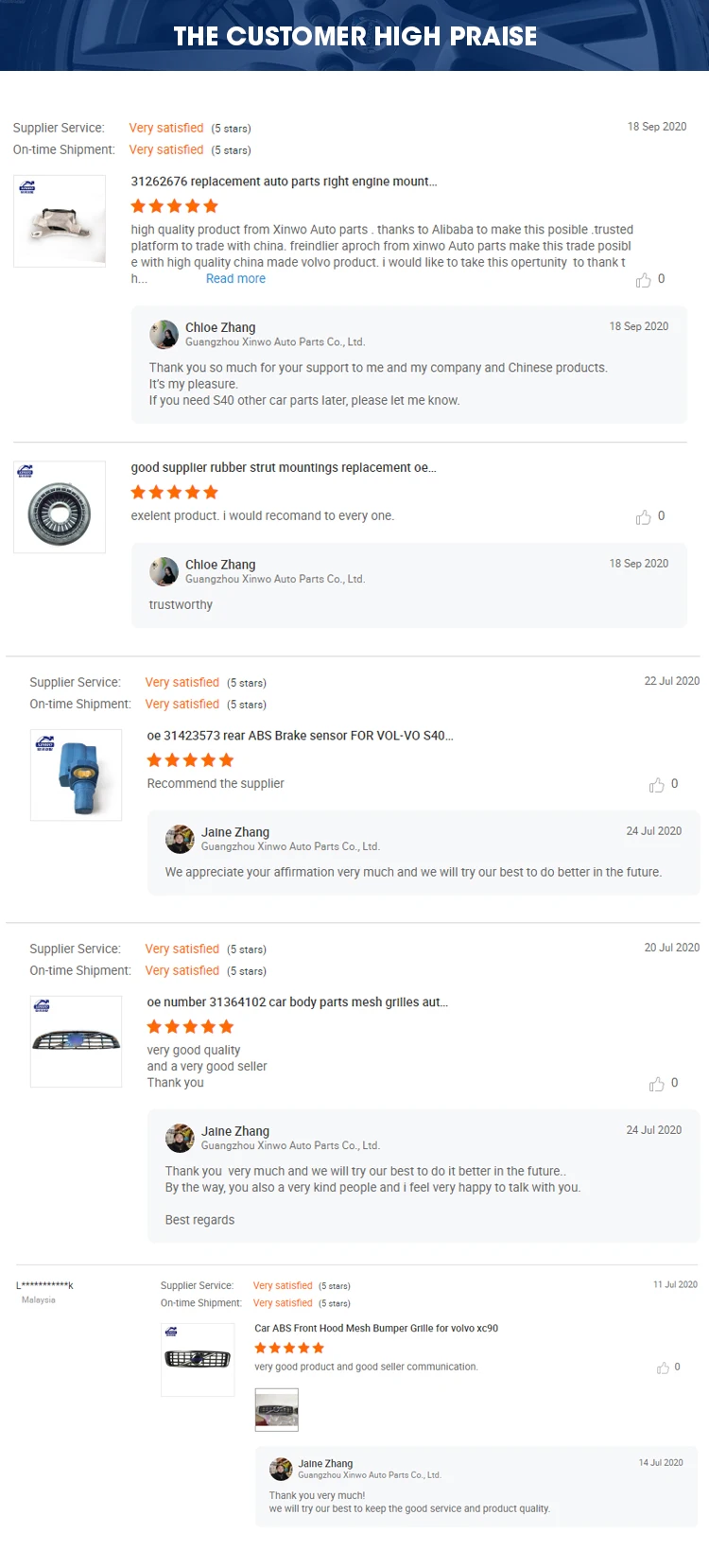**Detailed Image Caption: Customer Testimonials and Feedback for Guangzhou Zenvo Auto Parts Co., Ltd.**

At the top of the image, a blue grid pattern overlays the background of a tire. In bold, white, all-capital letters, the heading "CUSTOMER HIGH PRAISE" is prominently displayed. Below this, under the same blue grid pattern, the text "SUPPLIER SERVICE: VERY SATISFIED" appears in orange, accompanied by a five-star rating. Additionally, "ON TIME SHIPMENT: VERY SATISFIED" is also awarded five stars. The date "18 September 2020" is listed beside this review.

In the center of the image, a picture of the received auto part is shown. The text "31262676 REPLACEMENT AUTO PARTS" is visible alongside "5 STARS" and "HIGH QUALITY PRODUCT FROM ZENVO AUTO PARTS." Gratitude is expressed towards Alibaba, noting it as a "trusted platform to trade with China." The caption continues by praising Zenvo Auto Parts for its "brand new approach" and high-quality China-made Volvo product. It ends with "Read More" in blue, indicating there is more information available. Despite the many positive comments, a thumbs-up icon at the bottom shows zero likes.

Below, another feedback entry is featured with the title "GOOD SUPPLIER, RUBBER STRUT, MOUNTING REPLACEMENT, OE..." This review is rated five stars, labelling the product as "EXCELLENT" and highly recommended. A thumbs-up icon similarly shows zero likes. Guangzhou Zenvo Auto Parts Co., Ltd. responds on "18th September 2020," stating, "trustworthy."

A subsequent review underlines "SUPPLIER SERVICE: VERY SATISFIED" with a five-star rating, along with "ON TIME SHIPMENT: VERY SATISFIED" receiving another five stars. The title for this entry is detailed as "OE 31 4 2 3 5 7 3 REAR ABS BRAKE SENSOR, 4-S40..." dated "22, 2020," and awards five stars as a "RECOMMENDED SUPPLIER." Guangzhou Zenvo Auto Parts Co., Ltd. replies, expressing appreciation and a commitment to improve further.

Continuing, another five-star review highlights "SUPPLIER SERVICE: VERY SATISFIED" and "ON TIME SHIPMENT: VERY SATISFIED." This review's title reads "OE NUMBER 31 36 4 102 CAR BODY PARTS MESH GRILL IS AWESOME," dated "20 July 2020." The product is praised as having "VERY GOOD QUALITY" and the seller is acknowledged as very good. Guangzhou Zenvo Auto Parts Co., Ltd. responds with gratitude and a pledge to maintain high service and product quality.

The final segment of the image features a review attributed to "L****K, MALAYSIA," indicating "SUPPLIER SERVICE: VERY SATISFIED" and "ON TIME SHIPMENT: VERY SATISFIED." The review is for a "CAR ABS FRONT HOOD MESH BUMPER GRILL FOR VOLVO XC90," dated "11 July 2020," awarding five stars and commending the product and the seller's communication. Guangzhou Zenvo Auto Parts Co., Ltd. replies on "14 July 2020," thanking the customer and vowing to continue their good service and product quality.

Overall, the image showcases multiple reviews and positive feedback for Guangzhou Zenvo Auto Parts Co., Ltd., emphasizing their high-quality products, reliable service, and excellent customer relations.